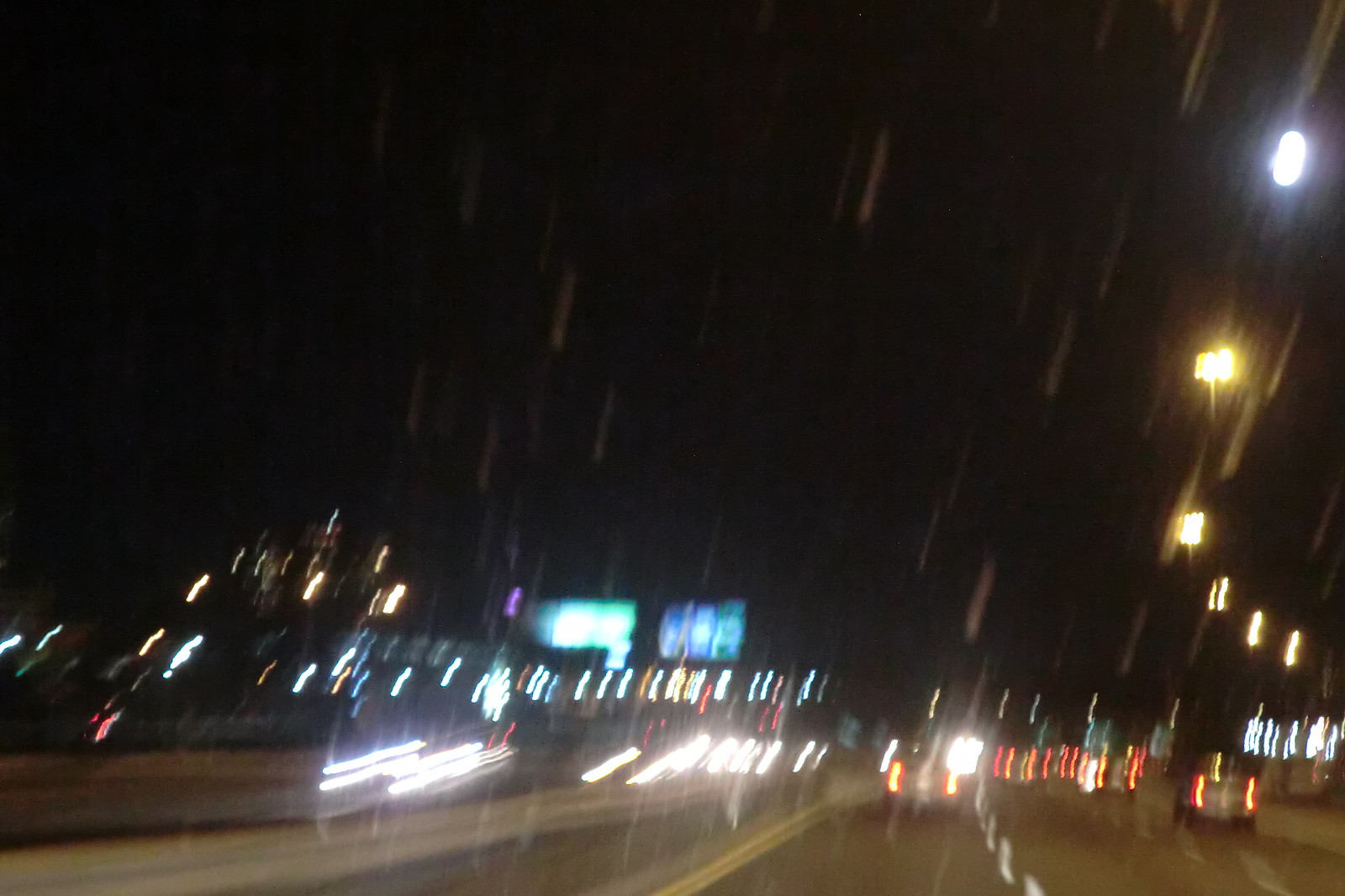A nighttime photograph taken from inside a moving car, looking through the rain-streaked window onto a well-lit, two-lane highway. The black top road is shimmering under the illumination of streetlights, reflecting the myriad raindrops that fall steadily. The car is traveling in the left lane, heading straight with no oncoming traffic on the opposite side. Several vehicles ahead can be seen, their taillights glowing a distorted, bright red due to the wet conditions and the motion of the car. Alongside the road, illuminated exit signs can be spotted, though their exact details are blurred and indiscernible in the darkness. The entire scene captures the quiet intensity and isolation of a rainy night drive.